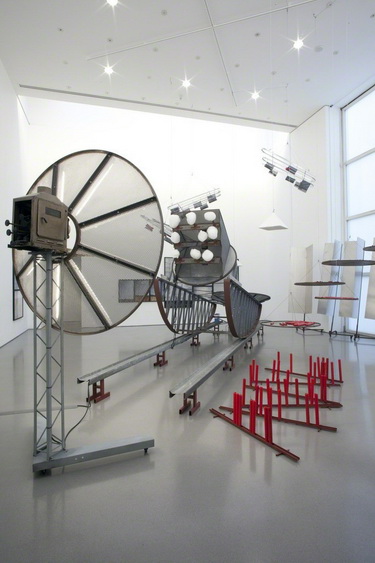The photograph depicts a well-lit white room, possibly a movie or recording studio, with a variety of unique structures and lighting arrangements. The ceiling features several cut-out lights that resemble stars, enhancing the room's brightness. On the right side, large windows provide additional natural light. 

In the center of the room, the principal structure consists of metal rails supporting a device with a unique eye-shaped wheel and a main piece adorned with numerous white dots or circles. This device, appearing to move along the tracks, has the outline resembling a boat and is designed to rock back and forth.

Near this central piece, a circular structure, resembling either a satellite dish or a camera light ring, is mounted on a vertical silver pole, facing the rocking device. 

On the right, there are brown metal frames with red vertical pieces protruding from them and several rods on the ground. Additionally, four white objects lean against the wall.

Lastly, in the background, a light that vaguely resembles a small airplane hangs from the ceiling, amidst five other ceiling lights contributing to the room's illumination.